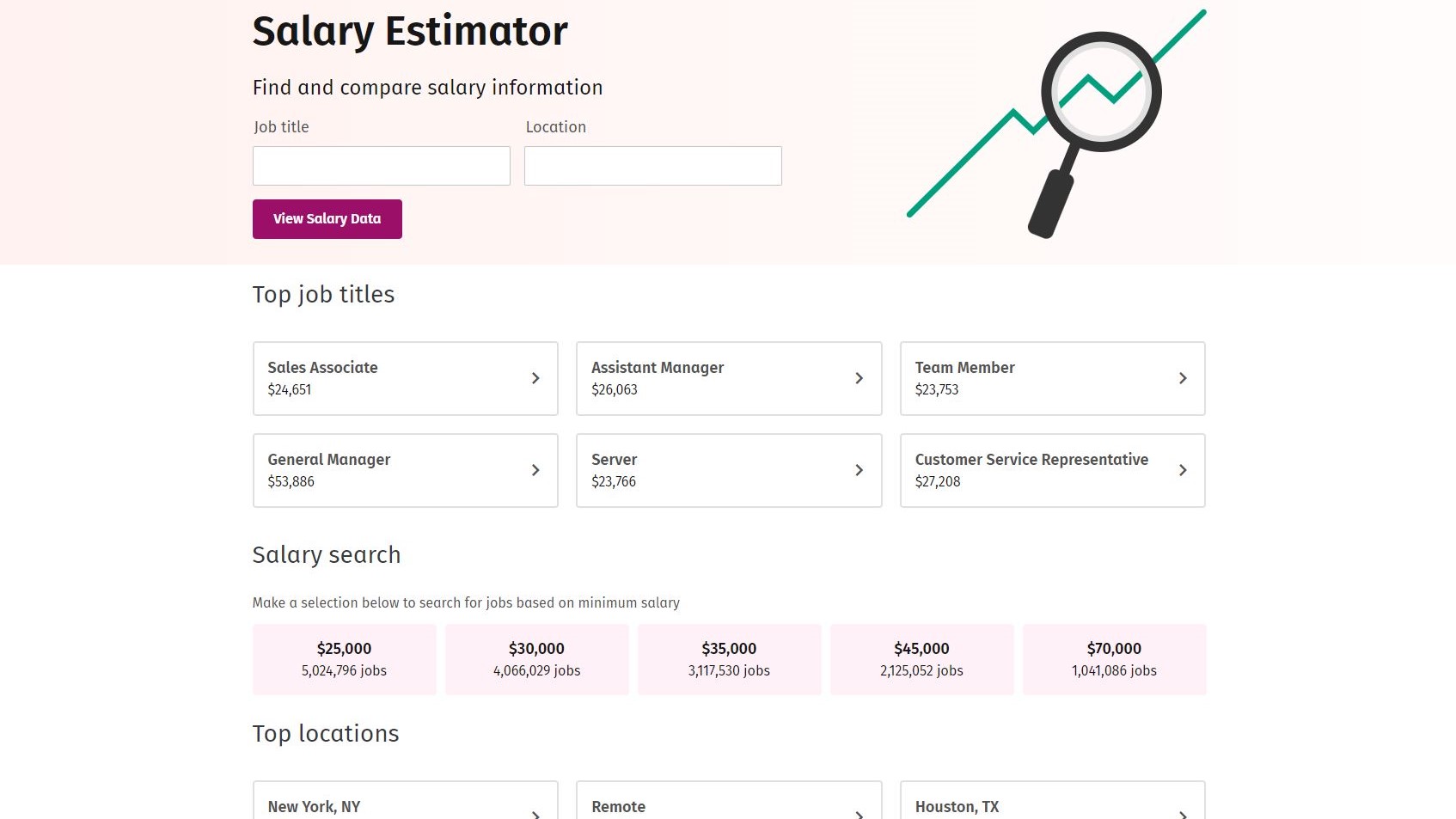This image, presumably from a website offering a salary estimator tool, features a well-organized interface with a distinct icon and vibrant color scheme. The prominent element is the icon situated in the top right corner, depicting a black magnifying glass focused on a green, upward-trending profit line, symbolizing increasing statistics against a soft pink background.

At the center of the interface, there are two text boxes. One stands out in fuchsia, labeled "View Salary Data," inviting users to interact with it. Adjacent to this, users can input their job title and location to "find and compare salary information." For instance, entering "Actress" as the job title and "Alaska" as the location prompts the tool to generate salary data.

Below these input fields, there are sections showcasing top job titles, each with corresponding salary figures. These are presented against a clean backdrop of white and black text, with the only additional color being the light pink background for selection points of the salary search. The first row includes:

1. Sales Associate: $24,651
2. Assistant Manager: $25,061
3. Team Member: $23,753

The next row, which includes clickable arrows for further details, features:

1. General Manager: $53,886
2. Server: $23,766
3. Customer Service Representative: $27,208

Further down, users can engage with the "Salary Search" feature by selecting a minimum salary range, with options like $25,000, $30,000, $35,000, $45,000, and $70,000.

Additionally, users can explore top locations for job searches including New York, NY, Remote, and Houston, TX. The image effectively encapsulates the functionality of the salary estimator tool, reflecting a user-friendly and visually appealing design.